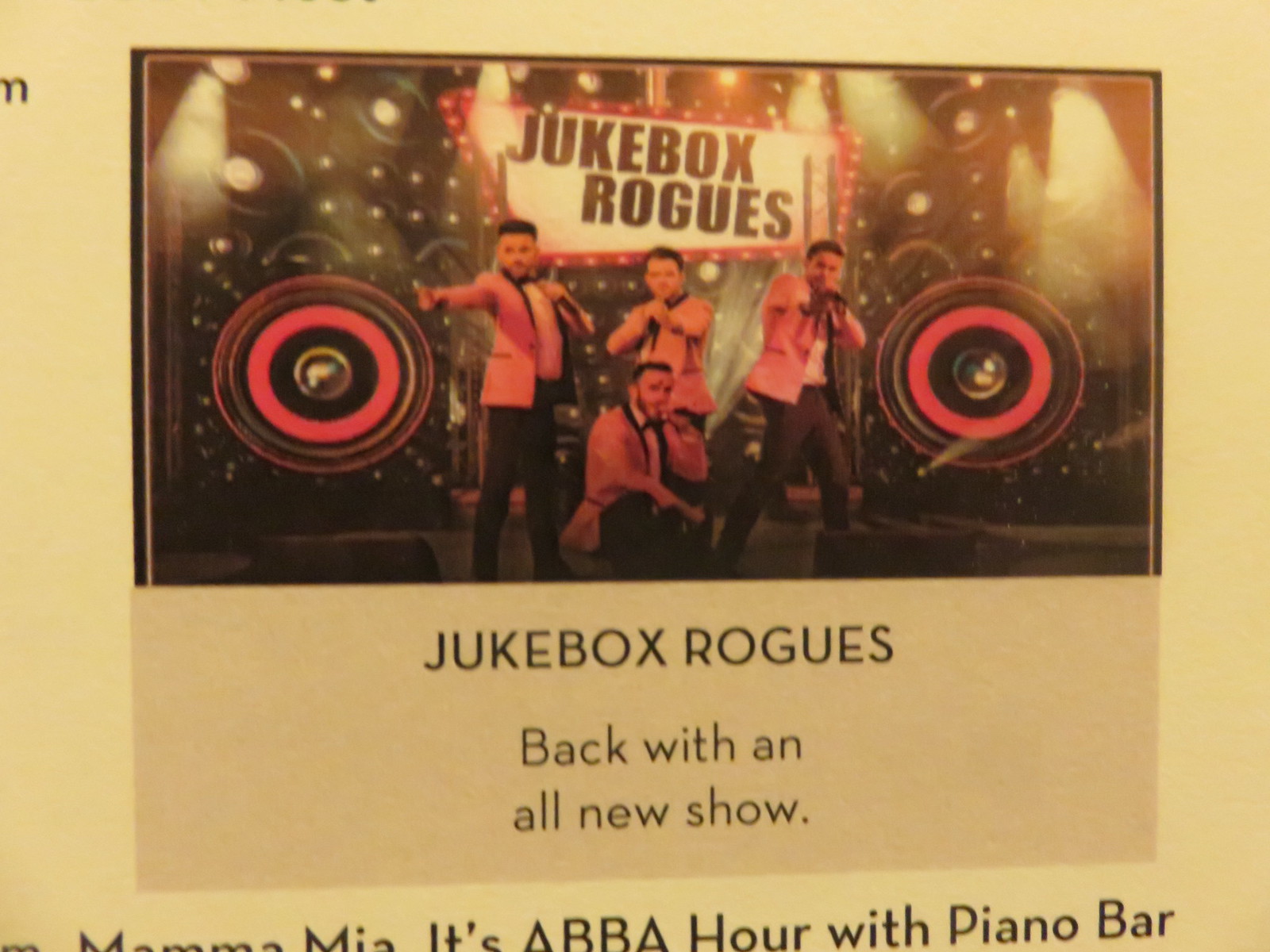The image is a slightly tinted, warm-toned photograph of an advertisement printed on white paper, possibly suffering from poor lighting conditions. It features a group of four men dressed in 1950s or early 1960s attire—pink blazers with black lapels, white button-down shirts, and black slacks—each holding wireless microphones. Three men are standing, and one is squatting in front. They are posed in front of large, black amplifiers with pink speaker sections, contributing to a retro aesthetic. Above the group, in black text on a white background, the sign reads "Jukebox Rogues." Beneath the image, printed on a gray section, the text reiterates "Jukebox Rogues" in all caps, followed by the phrase "Back with an all-new show." Below this, though partially cut off, the text reads "Mamma Mia, it's ABBA hour with a piano bar." Additionally, there are speaker icons on both the left and right sides of the image, enhancing its musical theme.